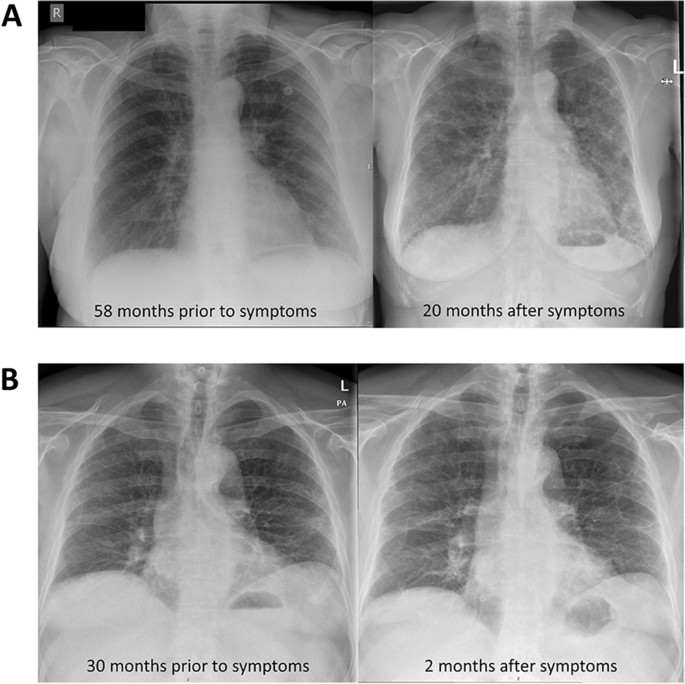This image displays a series of four chest x-rays arranged in two rows, labeled A and B, intended for educational purposes. Each row depicts the progression of changes in the lungs over different time intervals in relation to symptom onset. In row A, the first x-ray, taken 58 months prior to symptoms, shows clear lungs, predominantly black in color. The second x-ray labeled as 20 months after symptoms reveals noticeable white masses indicating abnormalities or disease within the lung tissues. 

Row B mirrors this format, but with different time intervals. The first x-ray in row B, labeled 30 months prior to symptoms, still shows relatively clear lungs with minimal white patches. The final x-ray, taken two months after symptoms, displays a significant increase in white masses within the lungs, coupled with a distinct black spot in the bottom right corner, highlighting a potentially critical development. The entire compilation of images underscores the progression of lung changes over time, moving from clear to increasingly obstructed with white masses, indicative of a condition affecting the respiratory system.